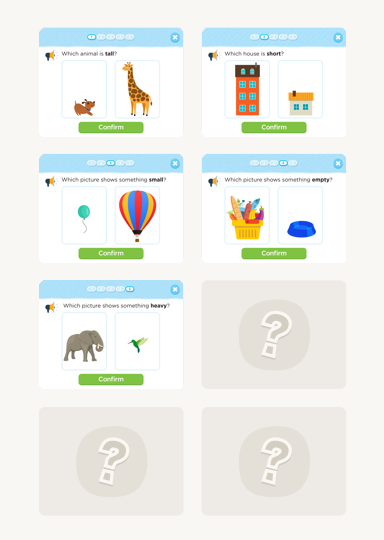The image displays a child's computer screen with a grid of eight boxes, each featuring interactive content designed to teach comparisons. The top row contains five frames with blue title bars and white backgrounds.

1. The first box shows a dog and a giraffe and poses the question, "Which animal is tall?"
2. The second box presents a tall house and a short house, asking, "Which house is short?" and includes a "Confirm" button.
3. Below the first box, on the left, there is a balloon and a hot air balloon with the query, "Which picture shows something small?"
4. To the right of that, the next box features a large basket full of food and a dog bowl, prompting, "Which picture shows something empty?" with another "Confirm" button.
5. Directly below, there is an image of an elephant and a hummingbird with the question, "Which picture shows something heavy?" and a green "Confirm" button.

Next to these, in the same row, is a single gray box with a white question mark in the center.

Beneath the gray box are two additional gray boxes, each containing a white question mark outlined in darker circles. The image is clearly part of an educational website designed to engage children with visually interactive and comparative questions.